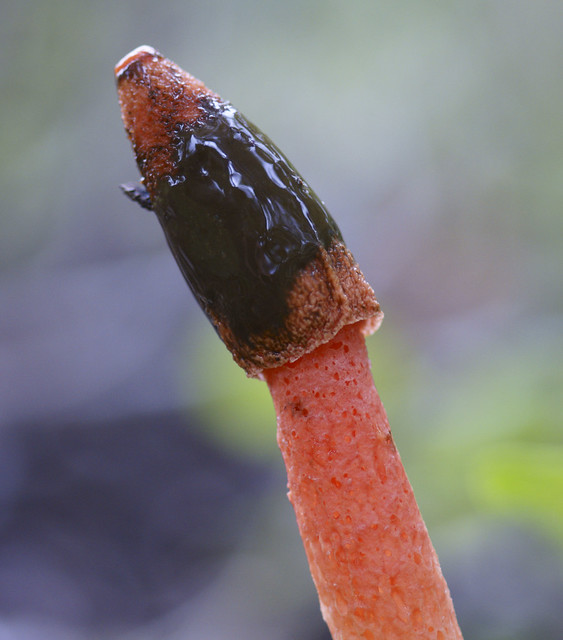The image displays a close-up of a peculiar pink branch-like structure extending towards the left, featuring a cone-shaped top. The branch's color is predominantly pink with various hue transitions, showing darker pink towards the top and sherbet-like tones near the bottom and left side. The top of the branch resembles a mushroom cap, characterized by a smooth, solid orange circular end. Just below this, the cap is adorned with a black, waxy liquid that encircles it, appearing glossy and reflective like old motor oil. Occasional orange spots with white speckles are seen amid the black liquid. The stalk of the structure is porous with darker openings or small holes, suggesting a less solid texture. Additionally, a screw-like feature with three lines is visible on the left side of the stalk. The background remains very out-of-focus, displaying vibrant hues of green, blue, and purple, with a bright neon green prominently on the bottom right side.